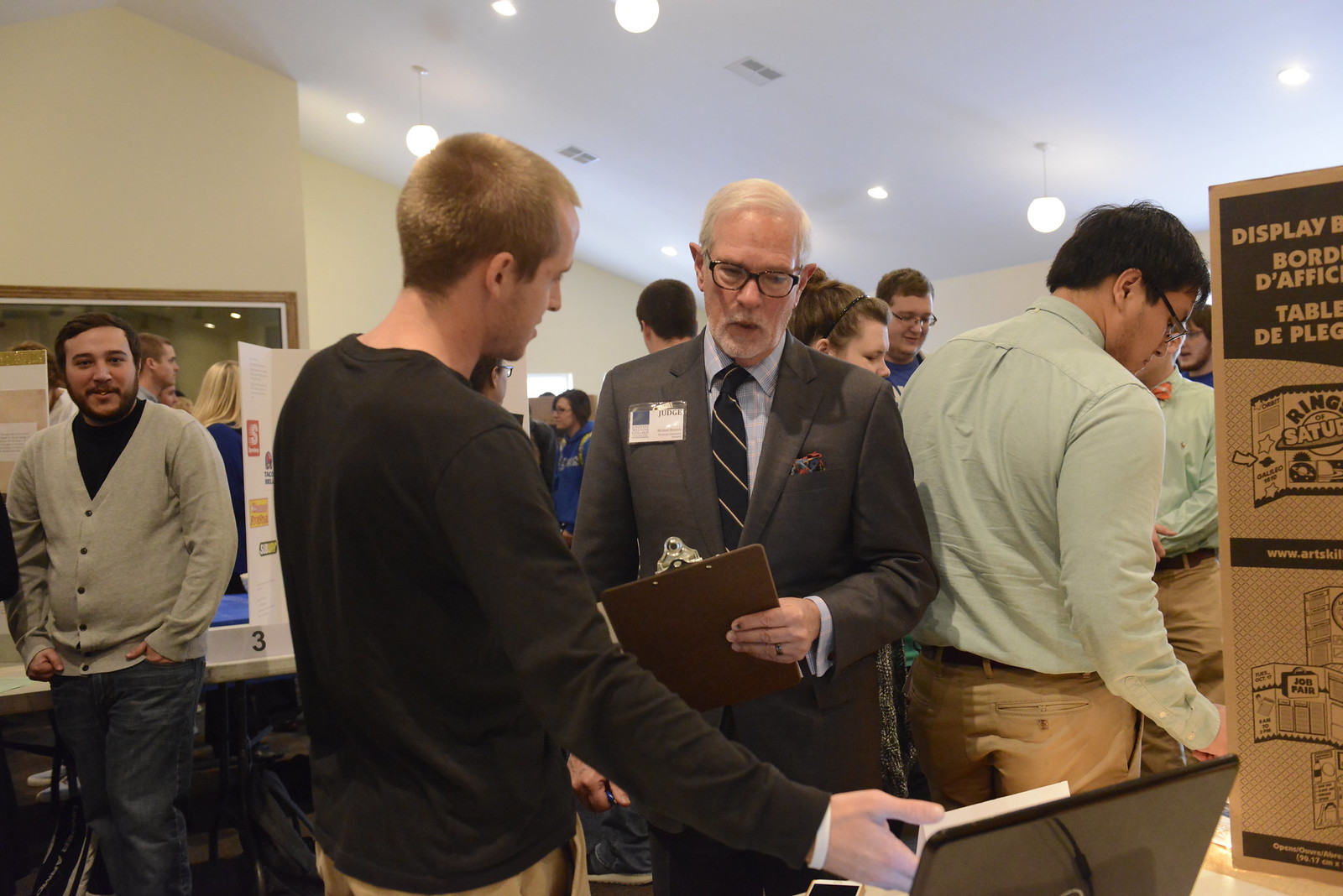In the image, a bustling seminar or technology event is depicted, featuring a group of predominantly young adults, many dressed in business casual attire. Central to the scene is an older gentleman, identified by his name badge as a judge. He is distinguishable by his white hair, white beard, glasses, and a conservative ensemble consisting of a suit, blue shirt, and a striped black tie. He holds a clipboard in his left hand and is focused intently on a laptop or tablet being pointed out to him by a younger man with short light brown hair, dressed in a long-sleeve black t-shirt, who has his back to the camera.

To the right of the judge, several individuals in mint green button-down shirts and khaki pants are visible, adding to the formal atmosphere. To the left, a casually dressed man stands out; he wears a white button-up sweater over a turtleneck and grey pants. His hands are in his pockets as he smiles and observes the interaction between the judge and the presenter. Additionally, a casually clad individual in blue jeans with a neat sweater and a turtleneck, who seems to be wearing a headset, watches the ongoing presentation attentively from the far left.

The room’s aesthetic is modest with tan-colored walls and a white ceiling, featuring around four hanging lights that illuminate the scene. In the background, other attendees are visible, mingling and engaging in discussions, contributing to the dynamic and engaged environment of the event.